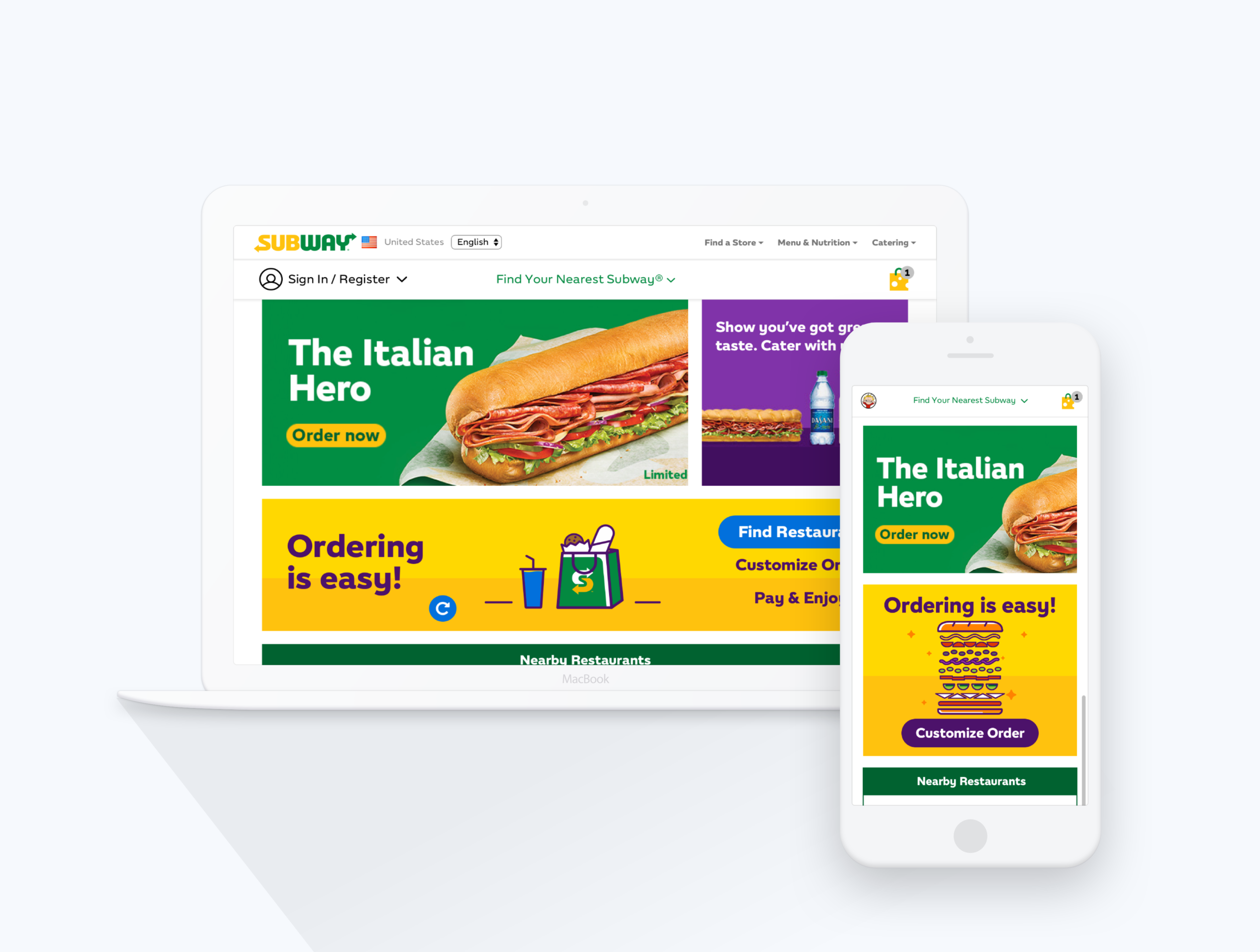The image features a detailed advertising layout for Subway, presented on a website with a light gray or blue square border. There are two main components showcasing the ad: one displayed as a webpage and the other as a mobile phone screen.

In the background, the webpage is in a rectangular, landscape orientation. The top prominently displays the word "Subway," with "Sub" in yellow and "Way" in green, accompanied by "United States" next to it. To the right, navigation options include: "Find a Store," "Menu," "Nutrition," and "Catering." Below these options, there is a "Sign In/Register" section, a "Find Your Nearest Subway" feature, and a shopping cart icon.

Centrally, the webpage highlights a green rectangular banner promoting "The Italian Hero" sandwich, with an appetizing image of the hoagie. Adjacent to it, a message invites users to "Show you've got great taste, cater with Subway," with visual elements including another hoagie and a bottle of water. At the bottom, a yellow rectangular border features text in purple stating, "Ordering is easy," beside illustrations of a bag and a drink. Directions for the user include: "Find a restaurant," "Customize order," "Pay and enjoy," and a green "Nearby Restaurant" button.

In front of the webpage mockup, there is a representation of a phone displaying the same Subway ad, formatted to fit a portrait orientation screen. This mock phone displays all the elements described on the webpage but rearranged to suit the vertical layout.